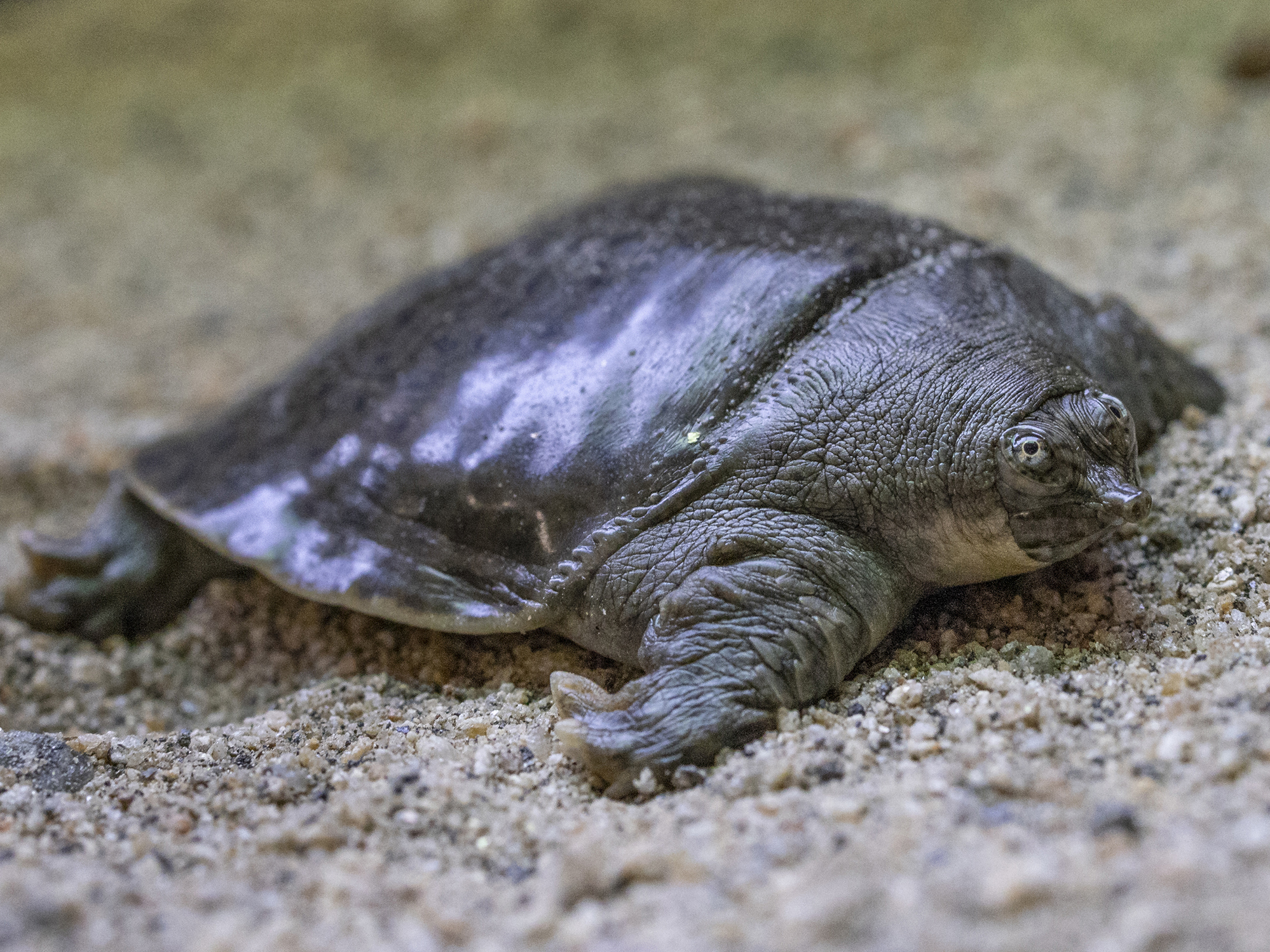This detailed wildlife photograph captures a distinctive gray soft-shell turtle on a light gray sandy surface. The turtle, approximately the size of a person's hand, features a smooth, leathery-looking shell that lies flat against its body, different from the typical hard, rounded shells of other turtles. The turtle's flipper-like legs are visible, with one arm and leg clearly seen on its right side. Its head, partly withdrawn into its neck, showcases a small, narrow snout with little nostrils at the end and bright, beady green eyes. The sand grains beneath suggest a small size for the turtle, and the blurred background emphasizes the turtle as the focal point of the image, with no additional text or copyright markings present.